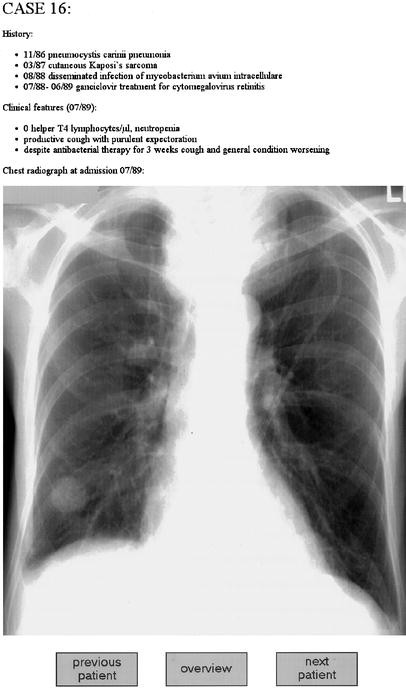The image reveals a worn and slightly aged x-ray from 1989, showcasing a rectangular view of a patient's lungs and ribcage. The ribs and lungs are dark in contrast to the predominantly white background of the body, with the area between the ribcage appearing completely white. Text at the top of the x-ray reads "Case 16: History" followed by several illegible scientific terms and dates, including references to conditions like pneumocystitis and sarcoma. Below this text, another section titled "Clinical Features (07/89)" lists symptoms such as zero helper T4 lymphocytes and a worsening cough despite antibacterial therapy. The x-ray is titled "Chest Radiograph at Admission (07/89)" just above the image displaying the ribcage in detail. At the very bottom, there are three navigation buttons labeled "Previous Patient," "Overview," and "Next Patient."